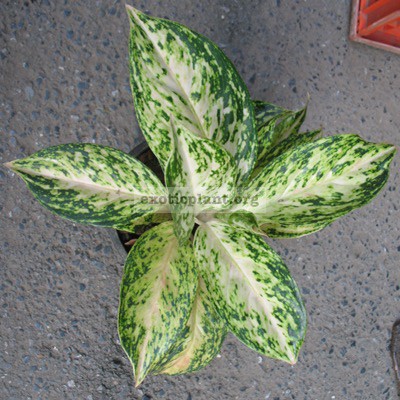The image depicts a top-down view of a potted plant, which takes up the majority of the frame. The plant is characterized by its large, speckled green leaves with cream-colored centers that fade into the green edges. There are about six to eight leaves visible, with larger leaves at the bottom and smaller, younger leaves growing from the top. The circular pot, which appears to be black, is partially visible, and the brown soil can be seen within it. The plant is placed on a gray speckled surface, with darker gray rocks embedded in it, suggesting a cemented or gravelly floor. In the top right-hand corner, a red column or similar object can be seen rising from the ground. Additionally, the image has a watermark in the middle that reads "exopicplant.org."